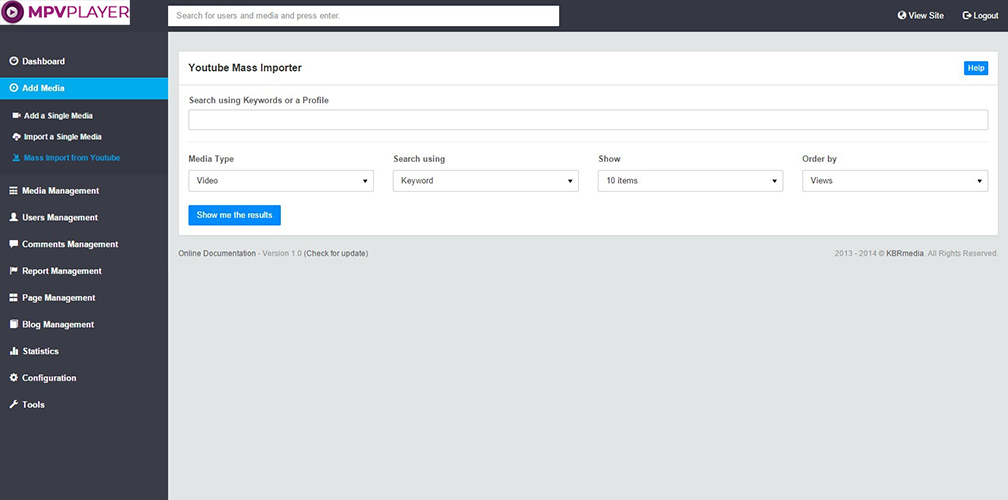This screenshot captures the interface of the mpvplayer software. The top left corner prominently features the mpvplayer logo, which is designed as a purple circle with a right-pointing rectangle and the text "mpvplayer." 

Running vertically down the left side of the screen, the dark grey menu bar is populated with a combination of white and blue text for easy readability. The larger, main pane displays a white and grey theme, dominated by the heading "YouTube Mass Importer."

Below this heading, users are prompted to perform a search using keywords or by selecting a profile, facilitated by a clearly visible search bar. Adjacent to this, a drop-down menu allows for the selection of the media type to search for, while another drop-down menu lets users specify the number of items to display. Additionally, there is an option to adjust the order of search results.

Upon configuring the search criteria, users can click on a blue button located at the bottom left-hand side labeled "Show Me The Results" to initiate the search. For user assistance, a small blue rectangle labeled "Help" is positioned in the top right corner of the interface.